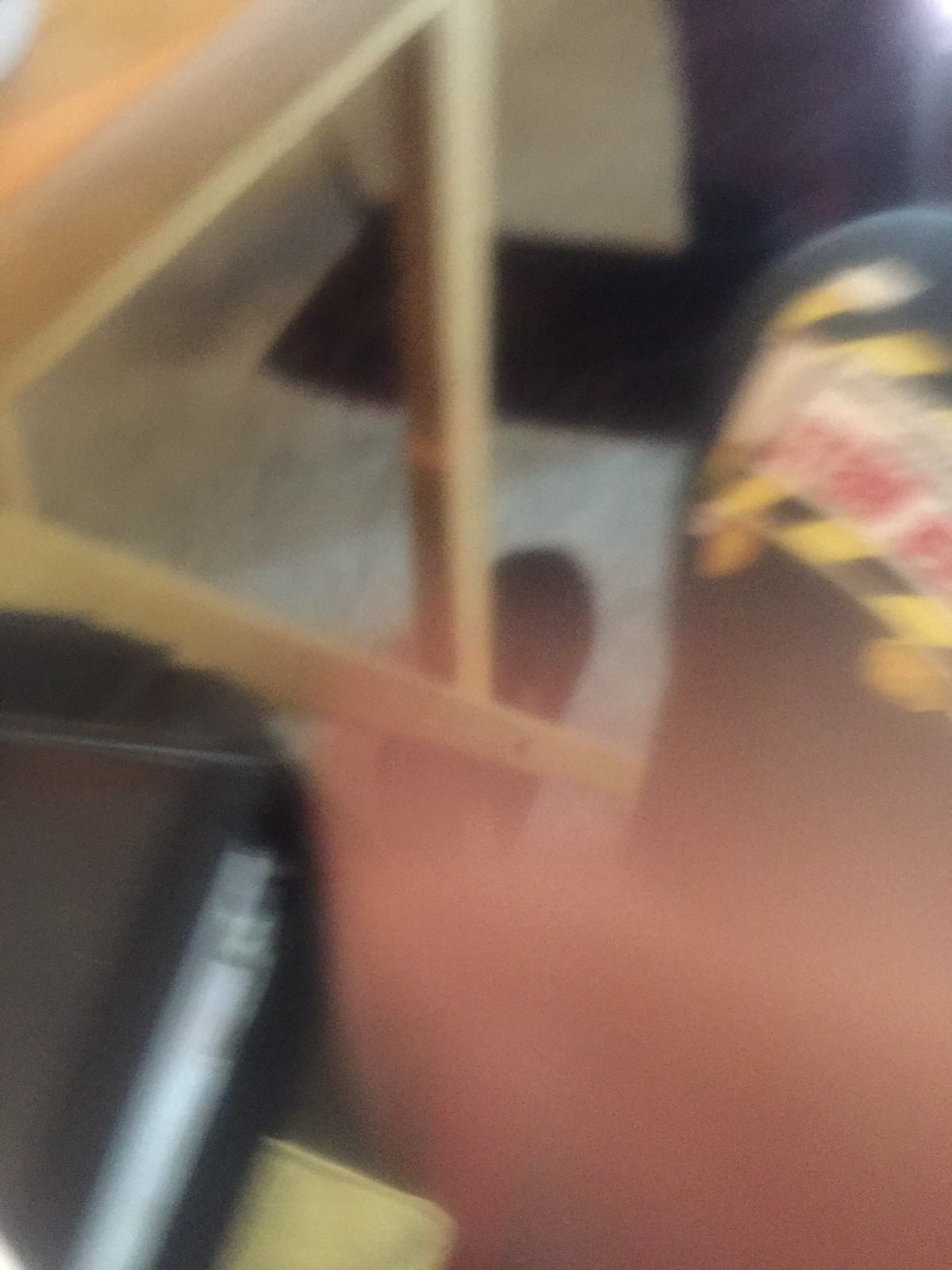The image is a vertically oriented, blurry photograph taken in a stairwell. Dominating the center of the picture is a yellow railing that runs diagonally from the bottom left to the upper right. Slightly off-center to the right, we see what appears to be the back of a man, though it's difficult to distinguish due to the blur. This figure is clad in black with a distinctive rectangle that features black and yellow coloring, possibly a logo, along with some illegible text in the center of the rectangle. At the bottom left corner of the image, there is a black binder resting on a surface, which might be another yellow binder, a seat, or even a step—it's hard to definitively tell. In the upper right background, a black door is faintly visible. The ground is a mix of gray and white, adding to the overall muted and unclear quality of the photograph.